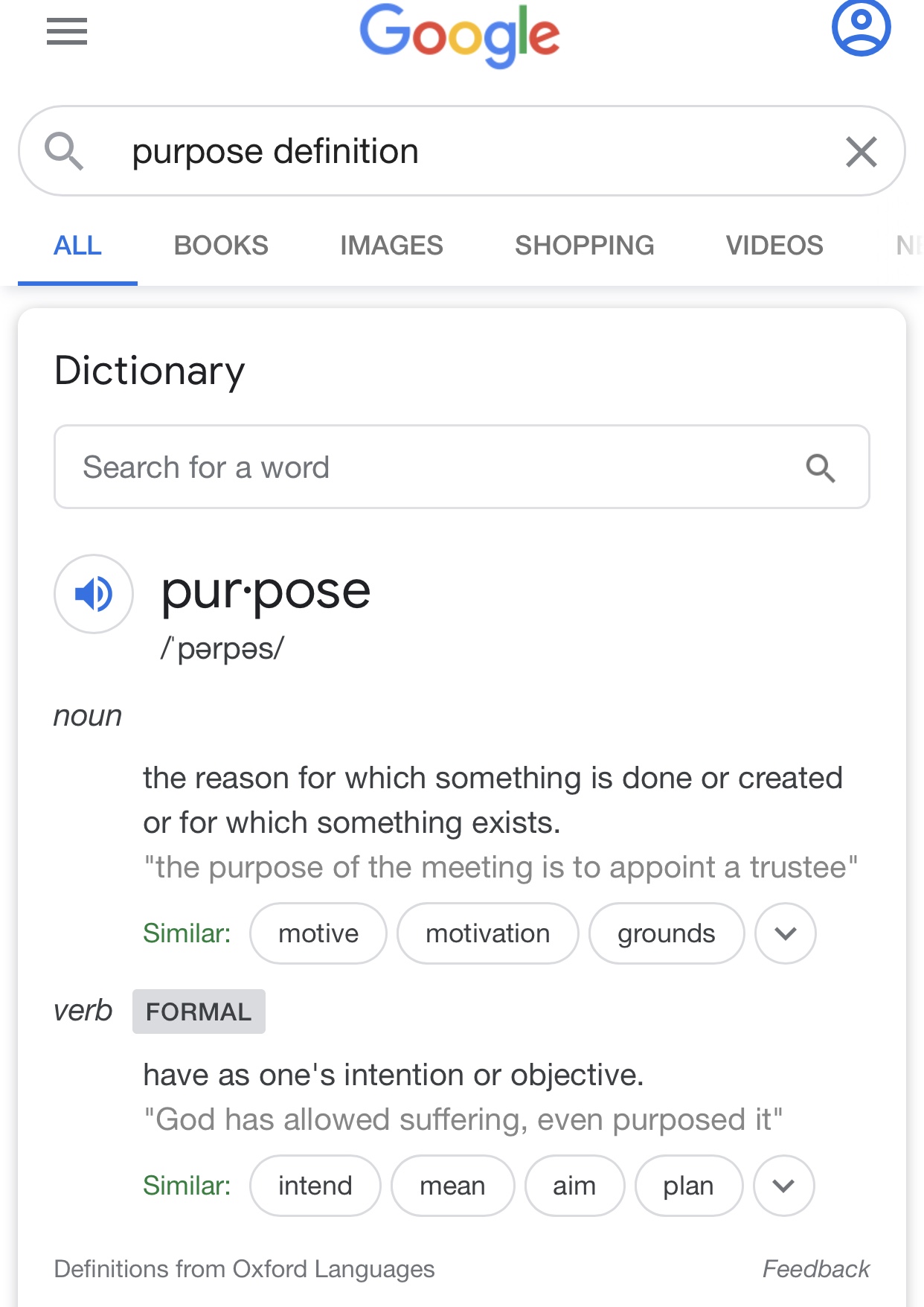Screenshot from a Mobile Device Displaying a Google Search for "Purpose"

The image is a clear and organized screenshot taken from a mobile phone or tablet. Central to the top, the familiar Google logo is presented in colorful lettering. To the left of the logo, there is a black "hamburger" menu icon, while on the right, a blue-edged circle contains a generic head and shoulders silhouette, representing the Google account icon.

Beneath the logo lies a search bar, which currently holds the text "purpose definition" indicating the user's search query. Below the search bar, multiple filter tabs are visible, specifically: "All," "Books," "Images," "Shopping," and "Videos," with the "All" tab selected.

Following this, there is a grey-edged rectangular section featuring an entry from a dictionary. At the top of this section, the word "dictionary" is prominently displayed, signaling the beginning of a detailed word analysis. The word in question is "purpose," and beside it, a blue voice icon allows users to listen to the pronunciation.

The word is initially identified as a noun. Its definition is provided as "the reason for which something is done or created, or for which something exists." An example sentence follows in grey italicized text: "The purpose of the meeting is to appoint a trustee." The section continues with a list of synonyms highlighted in green, including "motive," "motivation," and "grounds."

The entry then transitions to the verb form of "purpose," marked by a grey label indicating its formal usage. The definition here is "to have as one's intention or objective," with the example sentence: "God has allowed suffering, even purposed it." Synonyms for this usage include "intend," "mean," "aim," and "plan." Each list of synonyms is followed by down arrows indicating expandable lists.

At the bottom of the dictionary entry, the source is cited as "Definitions from Oxford Languages," with an option to provide feedback located on the right-hand side of the screen.